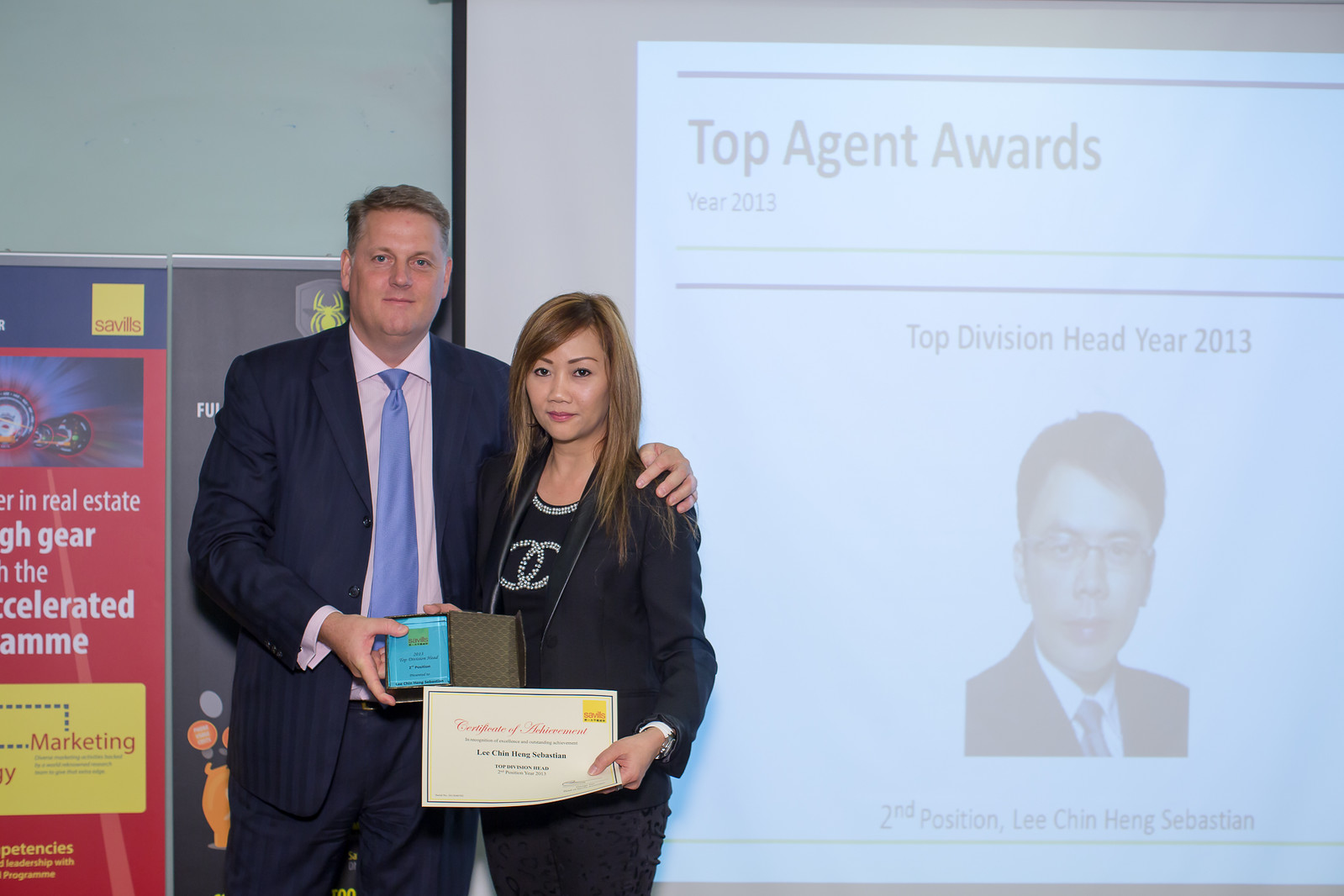In the photograph, which is shot indoors with a rectangular orientation wider than it is tall, a notable award presentation is occurring. At the center left of the image stands a Caucasian man in his late 40s, dressed sharply in a navy blue suit with subtle vertical stripes, a pink collared shirt, and a light blue tie. He has his left arm warmly around an Asian-descended woman, who has straight brown hair draping past her shoulders. The woman is elegantly attired in a black suit jacket over a black shirt adorned with rhinestones.

The gentleman holds a blue award in his right hand, which the woman also grasps, symbolizing the passing of recognition. In her left hand, she proudly holds a white certificate of achievement. Both individuals are intently looking at the camera, likely anticipating a photograph to capture this moment of acknowledgment.

Behind them, two significant elements frame the backdrop. To the left stands a green wall with a visible red banner partially reading, "Gear of the Accelerated Program." To the right, a white projection screen displays a slide in blue print, announcing the "Top Agent Awards Year 2013" and "Top Division Head Year 2013." Below these titles is a portrait of an Asian man, captioned "Second Position: Lee Chin Heng Sebastian." The scene suggests a formal recognition event, celebrating the accomplishments of top agents within the organization.